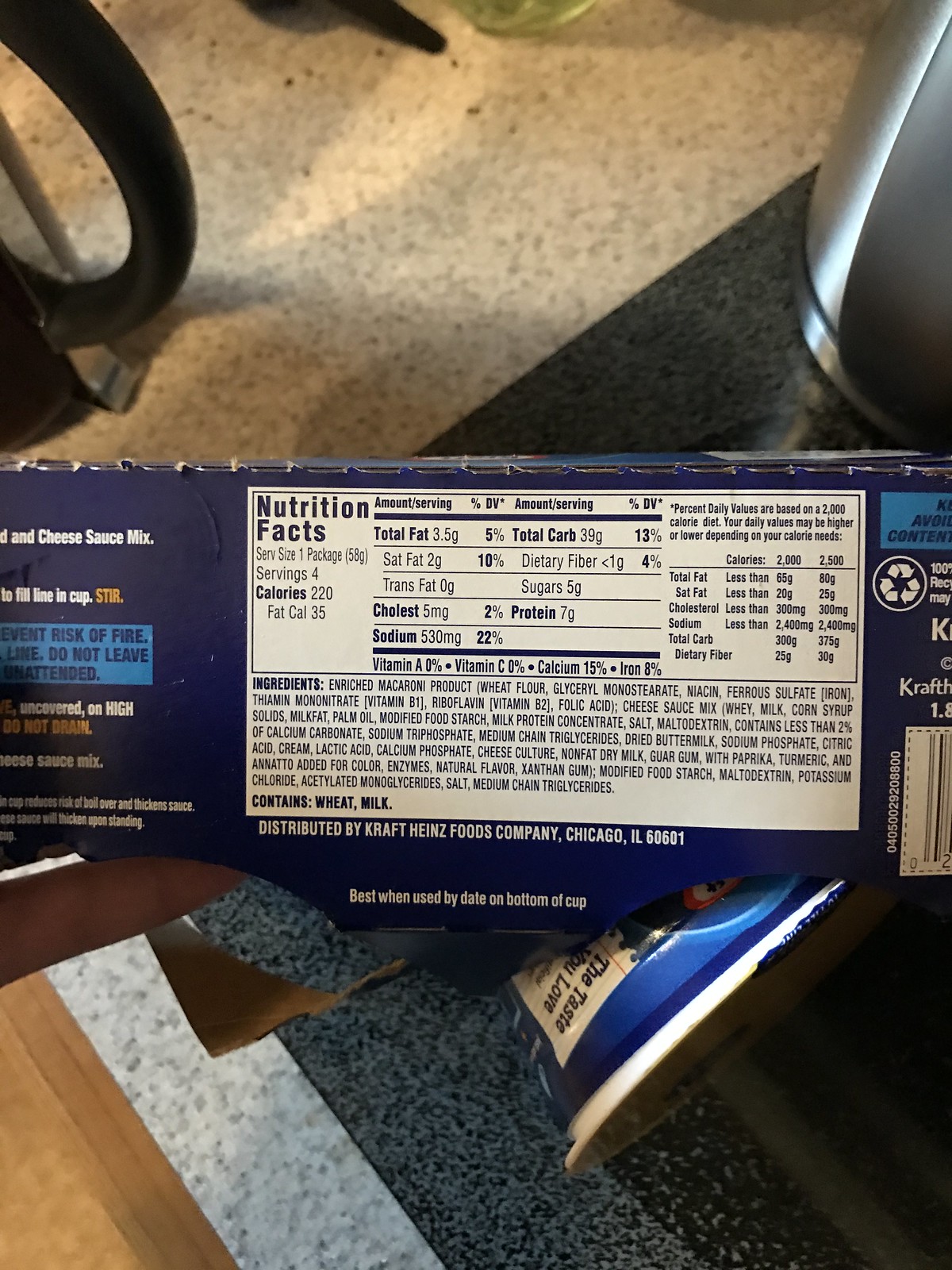The image depicts a vertical rectangular frame featuring a Kraft macaroni and cheese box positioned at an angle, displaying its label prominently. The box, dark blue in color, is situated on what appears to be the corner of a table or counter. Notable details visible on the box include the nutritional facts section, with key information such as "four servings" and "220 calories, fat calories 35," all printed within a white rectangular label. The label also mentions "cheese sauce mix" in white text and that the product is distributed by Kraft Heinz Food Company, Chicago, Illinois 60601. Additionally, the iconic "Kraft" logo is visible on the right side of the box, further confirming the brand identity.